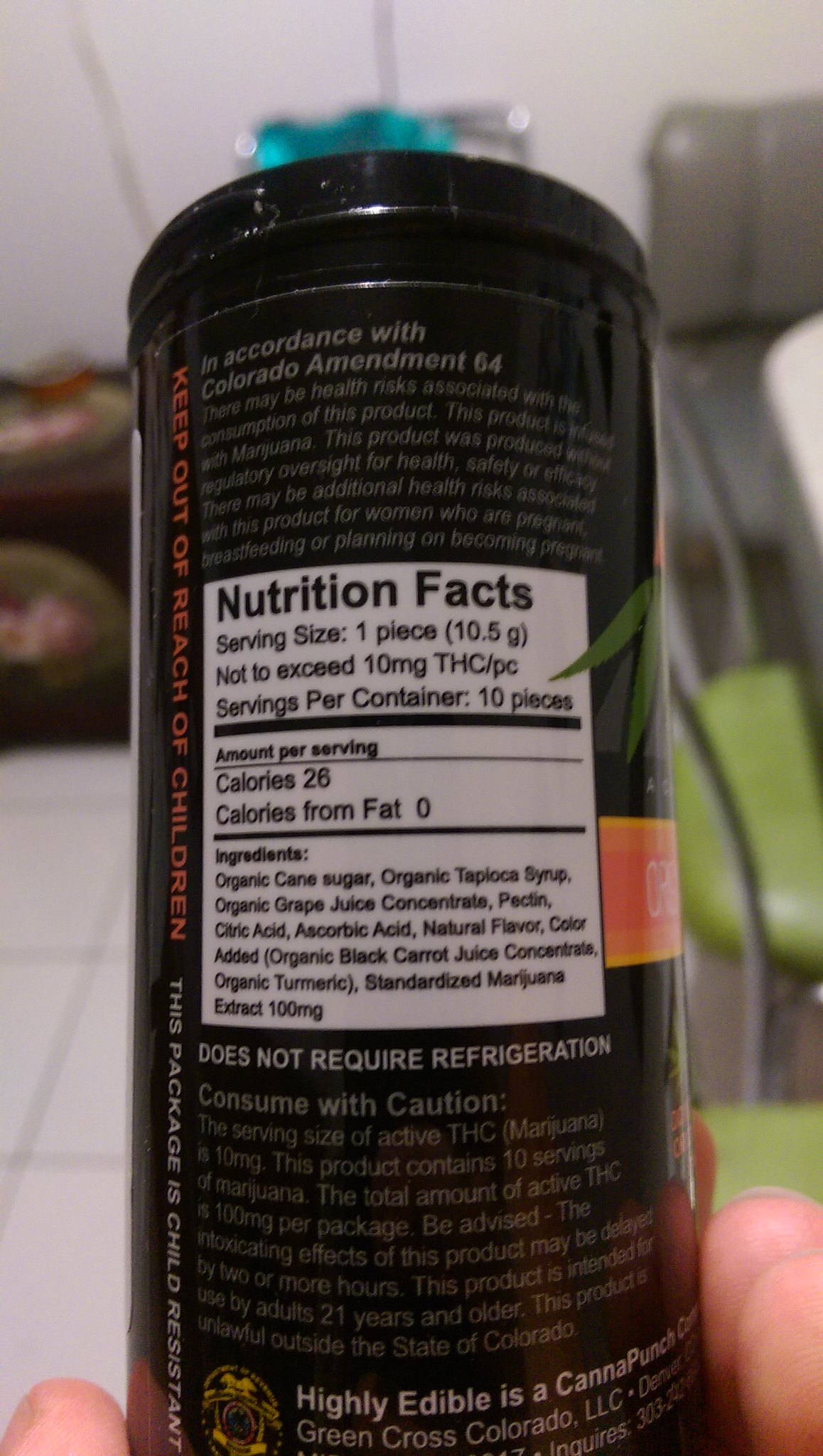In the rectangular image, we see a detailed photograph of the back of a black bottle with a gold or yellow stripe on the front right edge. Prominently displayed on the back label are the nutrition facts and a health warning in accordance with Colorado Amendment 64, indicating potential health risks associated with consuming the product. The nutrition facts detail a serving size of one piece, not exceeding 10 milligrams of THC-PC, and state that there are 10 pieces per container.

The list of ingredients includes organic cane sugar, organic tapioca syrup, organic grape juice concentrate, pectin, ascorbic acid, natural flavor, color added, and standardized marijuana extract, totaling 100 milligrams. Additionally, the product is identified as "Highly Edible" and branded as "Canna Punch," emphasizing that it does not require refrigeration.

A human hand, visible only by the fingertips at the bottom of the image, is holding the container, providing scale and context to the photograph.